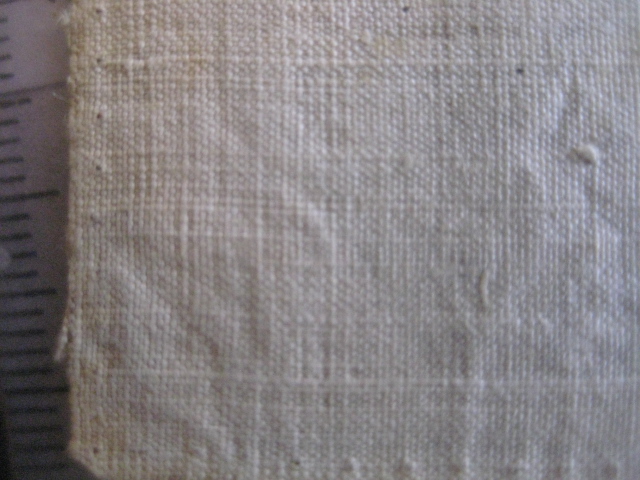The photograph features a close-up of a white woven material that appears to be a heavy cloth, possibly a grain bag or a tarp, characterized by its textured weave and small thread bumps forming a grid-like pattern. The fabric looks old, dirty, and possibly from an abandoned setting, suggesting it hasn't been cleaned in a long time. Along the left edge of the image, there are ruler-like lines without numbers, possibly indicating it's used for measuring. Additionally, there are sewing or needle holes around the edges, hinting at its previous use or repairs. The detailed texture and the aged appearance of the material make it unclear what its exact purpose is, but it evokes a sense of utility and history.